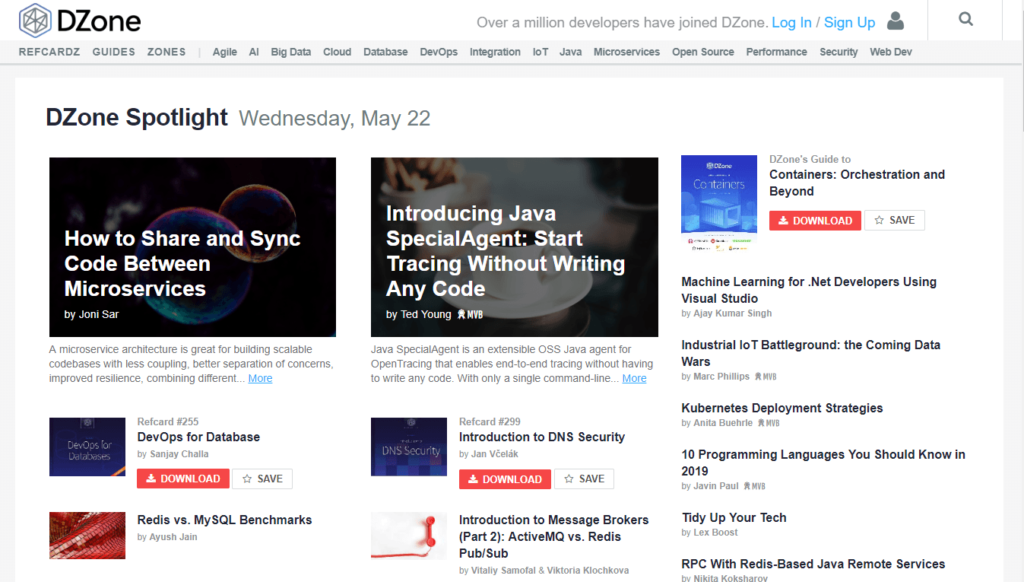Screenshot of the D-Zone website homepage:

In the upper left corner, the D-Zone logo stands prominently, featuring a hexagon within a hexagon design. Intersecting lines from corner to corner within the hexagon subtly form the letters 'Z' and 'N,' representing the name "D-Zone."

To the right of the logo, a prominent message declares, "Over a million developers have joined D-Zone." Adjacent to this assertion are login and sign-up hyperlink buttons, accompanied by a small figure icon, likely for user profiles, and a magnifying glass icon in the upper right corner, indicating the search function.

Below this header, a horizontal navigation bar spans from left to right, offering quick access to various sections:
- Ref Cards
- Guides
- Zones
A vertical separator follows, dividing the main categories from specific topics:
- Agile
- AI
- Big Data
- Cloud
- Database
- DevOps
- Integration
- IoT
- Java
- Microservices
- Open Source
- Performance
- Security
- Web Dev

Next, a section titled "D-Zone Spotlight" is displayed, featuring the date "Wednesday, May 22nd," followed by a selection of various articles.